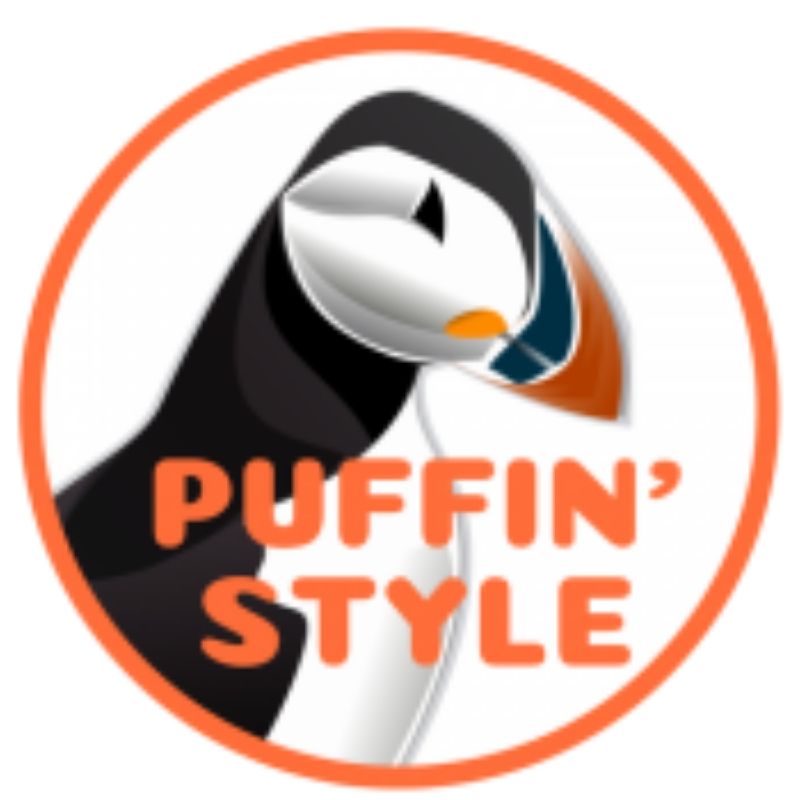This image features a stylized, geometric logo set against an entirely white background. Dominating the center is an orange circle reminiscent of the Dunkin' Donuts color palette, encapsulating the upper half of a bird resembling a puffin, though with penguin-like black and white coloring on its chest and back, and a vibrant blue and orange beak. The puffin is facing slightly downwards to the right, with a simple, minimalist design that is not photorealistic. Encircling the bird within the orange border, the text "PUFFIN' STYLE" is prominently displayed at the bottom third of the image in a matching orange, capitalized font similar to that of Dunkin' Donuts. The overall composition suggests it may serve as a company logo, with its clean, bold elements occupying the majority of the image space.